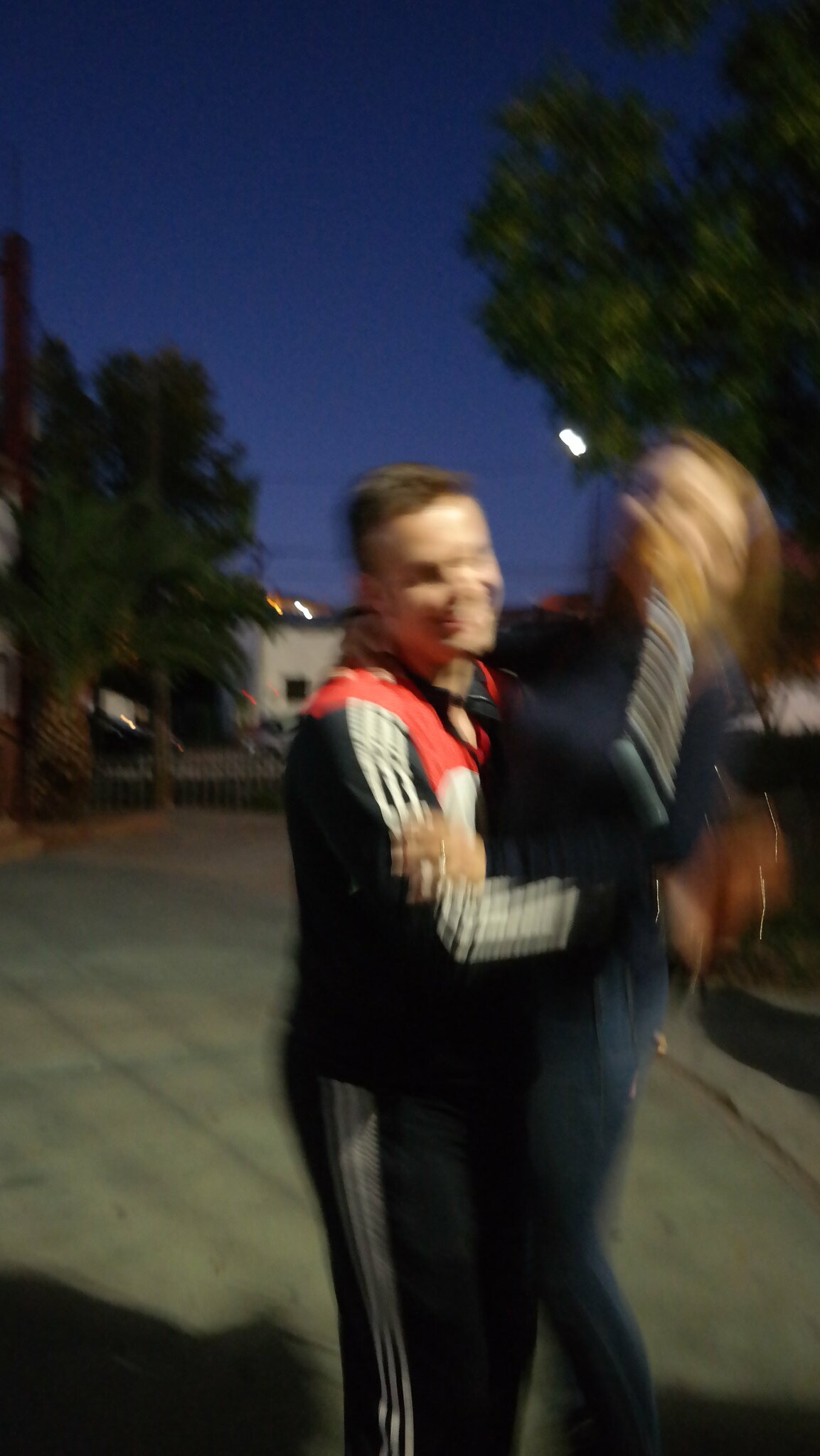In this somewhat blurred photograph, a couple is captured in the midst of what appears to be a joyful moment. The man, who is fair-skinned with short brown hair, is dressed in a black jogging suit featuring three white stripes running down the arms and legs. Beneath the suit, he wears a shirt with striking red and white colors. His broad smile is unmistakable, radiating happiness as he holds a woman close. The woman, though her face is even more blurred than his, can be seen wearing a blue sweater paired with blue jeans. A brown purse is slung over her shoulder, adding a casual yet stylish touch to her outfit. The blurriness of the image suggests motion, perhaps indicating that the couple is dancing or moving together, encapsulating a moment of shared joy and spontaneity.